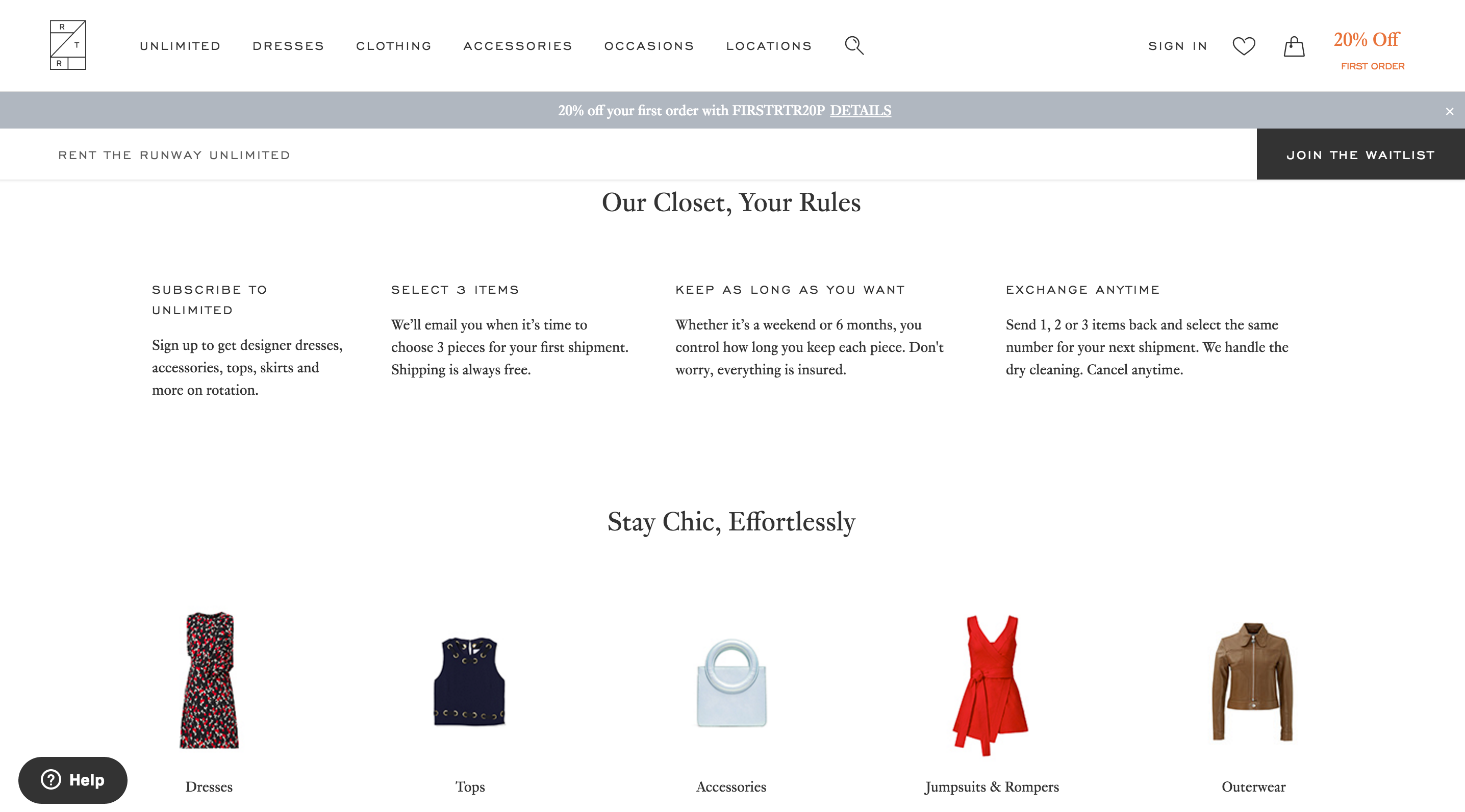This image is a screenshot of a fashion rental website. The topmost section features a white navigation bar containing various categories such as "Unlimited," "Dresses," "Clothing," "Accessories," "Occasions," and "Locations," along with a search bar. Adjacent to this are icons and links for "Sign-in," a heart symbol, a shopping bag, and a promotional message that says "20% Off Your First Order."

Below the navigation bar, there's a gray banner proclaiming "20% Off Your First Order" accompanied by the website's name, although the company name isn't legible. Another text just below this banner reads "Rent the Runway Unlimited."

In the central part of the page, the bold statement "Our Closet, Your Rules" is prominently displayed, with a call-to-action button labeled "Join the Waitlist" to the right. Further down, the text "Subscribe to Unlimited" is followed by a brief explanation of the service: "Select items. Keep as long as you want and then exchange anytime." Beneath this description, the phrase "Stay Chic Effortlessly" is seen.

The lower part of the screenshot features categorized images for different types of clothing and accessories. For "Dresses," there's an image of a colorful dress; "Tops," features a sleeveless top; "Accessories," displays a purse; "Jumpsuits and Rompers," showcases a picture of a red romper; and for "Outerwear," there's an image of a jacket. 

Overall, the background of the entire webpage is white, emphasizing a clean and streamlined aesthetic for this clothing rental service.